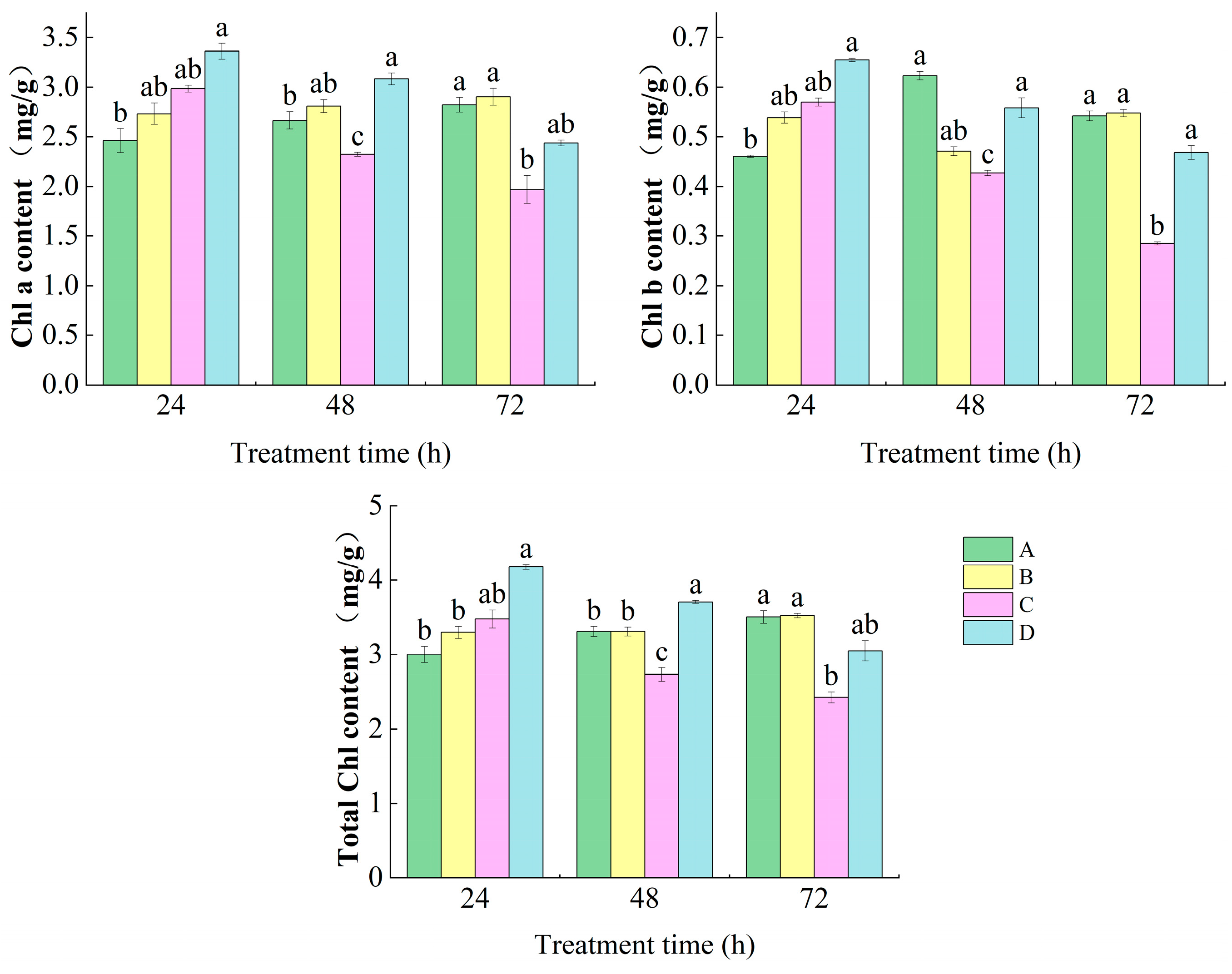The image displays a set of three detailed bar charts against a white background, illustrating the variations in CHLA, CHLB, and total CHL content over different treatment times, measured in hours (H). Each bar chart features columns in four distinct colors—green for A, yellow for B, pink (or mauve/purple) for C, and blue for D—demonstrating the respective contents in milligrams per gram (mg/g).

1. **CHLA Content**: The first bar chart shows the CHLA content, with the y-axis ranging from 0 to 3.5 mg/g, and the x-axis labeled as treatment time in hours, highlighting distinct intervals up to 72 hours.
2. **CHLB Content**: The second bar chart displays the CHLB content, where the y-axis spans from 0 to 0.7 mg/g, following a similar x-axis structure showing treatment times.
3. **Total CHL Content**: The final bar chart at the bottom illustrates the total CHL content, with the y-axis extending from 0 to 5 mg/g, again plotted against treatment times up to 72 hours.

All three charts consistently use green, yellow, pink, and blue to represent lines A, B, C, and D, respectively. This uniformity allows for a clear comparative analysis of content changes over specified treatment durations, potentially informing a scientific or medical study.